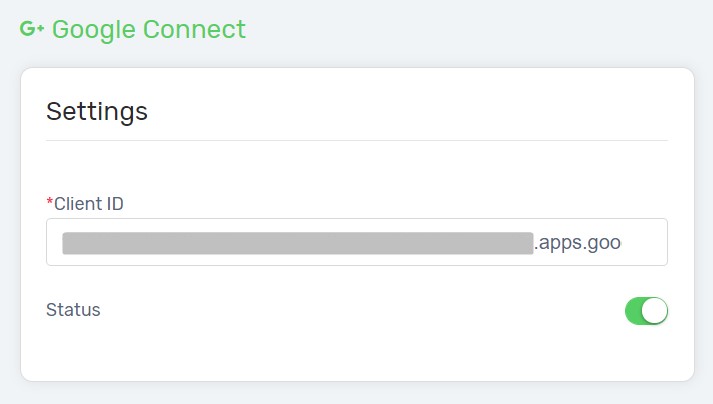This image is a detailed screenshot of a settings screen. The background is a pale grey, providing a neutral backdrop for the elements in the forefront. 

In the upper left corner, a small "G" with a green plus sign next to it is prominently displayed, indicating an addition. Adjacent to this icon, the text "Google Connect" is clearly written in bright green.

Centered below this heading is a white, landscape-oriented rectangle with rounded corners, creating a distinct separation from the background. Within this rectangle, in the top left corner, the word "Settings" is bolded in black and underlined with a thin grey line that extends horizontally across the rectangle.

Directly beneath "Settings," a red star indicates a mandatory field labeled "Client ID." Below this label is an input field, where most of the content has been redacted for privacy with a grey rectangular block. However, the edge of the redacted text reveals a partial URL, ending in ".apps.goo."

At the very bottom of this rectangle, the word "Status" is found in the bottom left corner. Contrastingly, in the bottom right corner, a toggle button for the status is switched to the "on" position, indicated by a green color. 

This careful arrangement and color scheme contribute to the functional and user-friendly design of the settings interface.